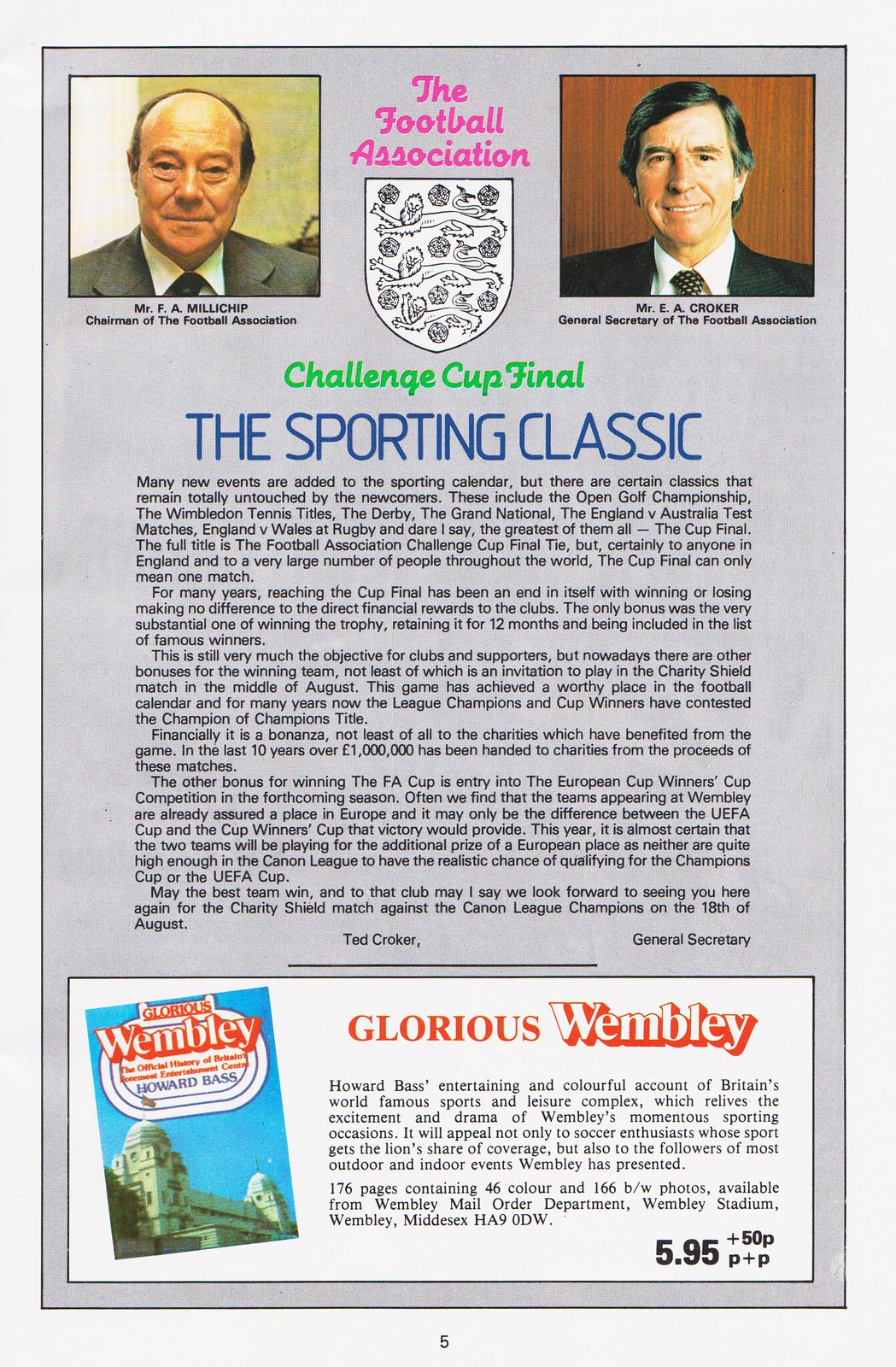The image depicts an excerpt from a pale purple leaflet or magazine page about the Football Association, prominently featuring the title in vibrant pink text above a crest that includes caricatured lions and possibly roses. On either side of the crest are photographs of two men in suits: Mr. F.A. Millichip, Chairman of the Football Association, on the left, and Mr. E.A. Croker, General Secretary of the Football Association, on the right. Large text below the crest announces the "Challenge Cup Final," followed by "The Sporting Classic" in blue font. The leaflet details the importance of the Cup Final, comparing it to other historic sports events like the Open Golf Championship and the Wimbledon Tennis Titles. A letter from Ted Croker mentions anticipation for the Charity Shield Match against the Canada League Champions on August 18th, although the year is not specified. The page, marked as number 5 at the bottom, also includes an advertisement for a book titled "Glorious Wembley," with purchase information. The entire layout features black text on a gray background.